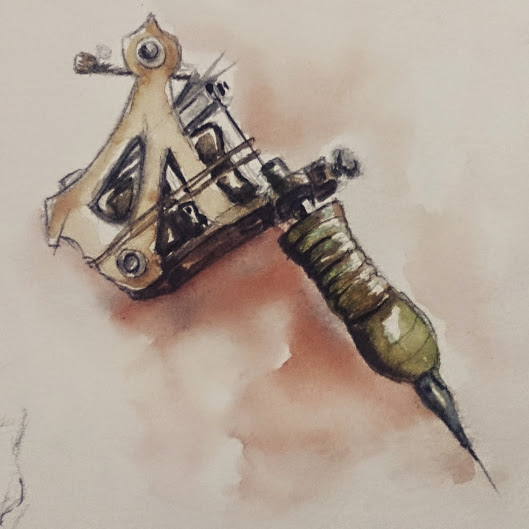This artistic rendering appears to depict a complex mechanical device, most likely a tattoo machine. The artwork is set against a white paper backdrop, marred by smudges of rust-colored hues, varying in intensity, likely intended to represent shadows cast by the apparatus. The machine's metallic structure is suggested by the depiction of numerous screws and mechanical details.

At the forefront, a prominent needle-like component is evident, hinting at its potential function. Accompanying this needle is a green ergonomic grip, seemingly designed for comfortable handling. Extending from this grip is a dark gray nib, suggesting a conduit for ink flow. The dark, intricate design gives the impression that black ink might be involved in its operation.

Connected to the main body of the device, there are additional elements that could possibly be ink reservoirs or containers, enhancing the overall intricacy of the machine. While the exact nature of this contraption remains ambiguous, its resemblance to a tattoo machine is strong, indicating it might be an artist's detailed interpretation of such equipment.